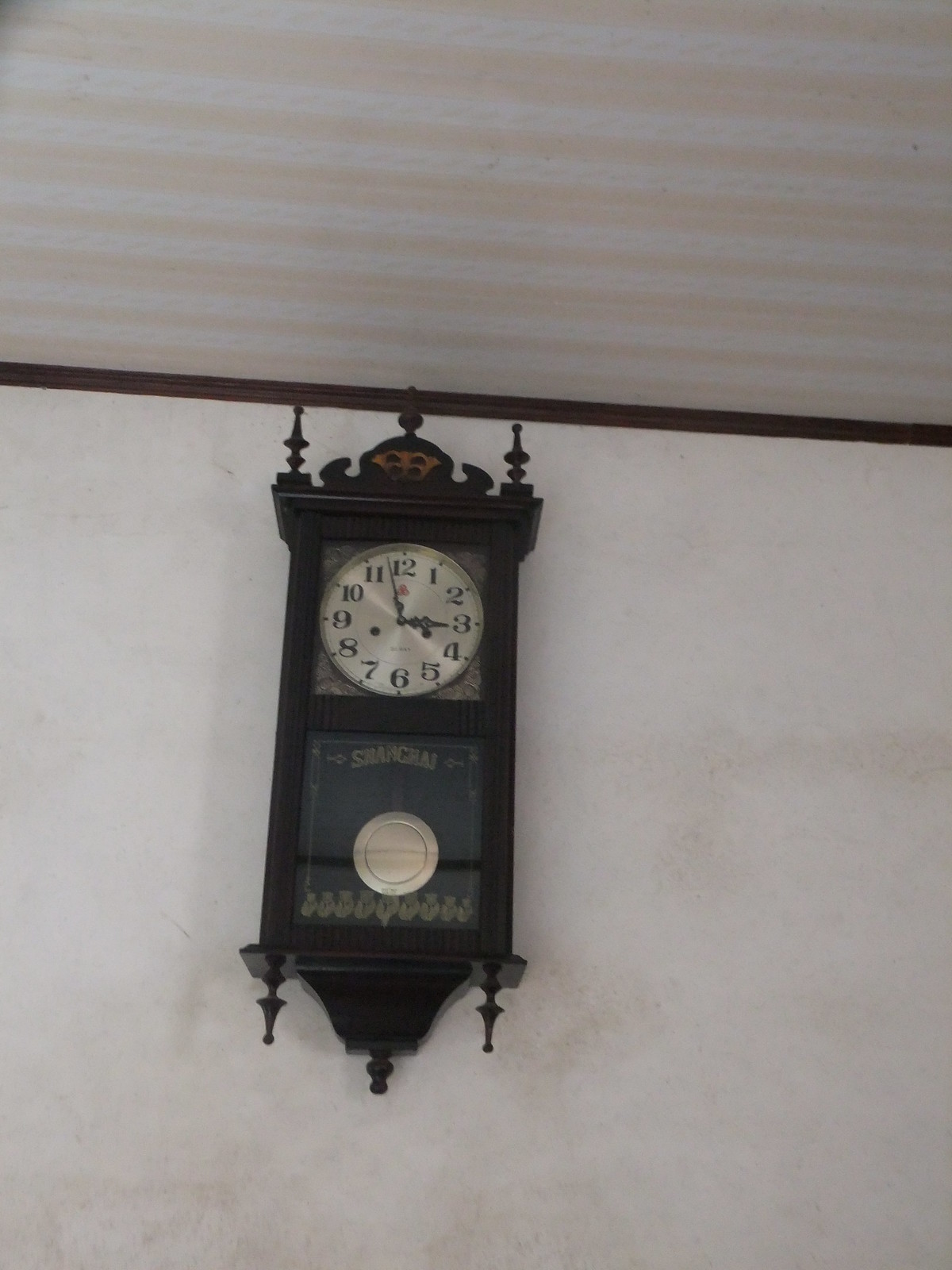This image portrays a dimly lit interior where the viewer's perspective is slightly angled upwards towards the ceiling, which occupies the upper third of the composition. The ceiling features distinctive horizontal stripes in subtle shades of light blue and peach. The border between the wall and ceiling is characterized by dark brown molding. The off-white wall serves as the backdrop for an ornate antique clock that is mounted high, just below the ceiling.

This intricate clock is framed in dark wood, with elaborate spires extending from its top and sides. The upper half of the clock showcases a silver face with black numerals and hands, indicating the time as 2:57. Below this, a pendulum dangles within a rectangular wooden structure. The combination of the striped ceiling, dark brown molding, and the detailed clock evokes a sense of vintage elegance in the room.